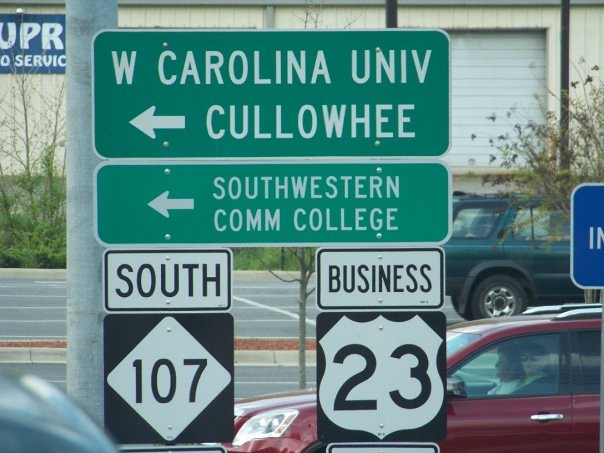This daytime photograph captures a busy urban intersection, with a multitude of street signs mounted on a silver metal pole in the foreground. The signs provide directions to various destinations. At the top is a green rectangular sign with white text, indicating "W. Carolina University, Cullowhee" with an arrow pointing left. Below it is a similarly styled green sign for "Southwestern Community College," also with a leftward arrow. At the base of the pole, there are two sets of route signs: the left set features a white rectangular sign labeled "South," above a black square with a white diamond and the number "107" in black. To the right of these, a white rectangle states "Business," which is positioned above a black square bearing a white U.S. highway shield with the number "23." In the background, a beige building with a large garage door and a white covering is visible, along with a red car and a dark SUV near a highway with a red stone divider flanked by concrete curbs. The road appears to be two to four lanes wide, capturing the bustling essence of the street scene.